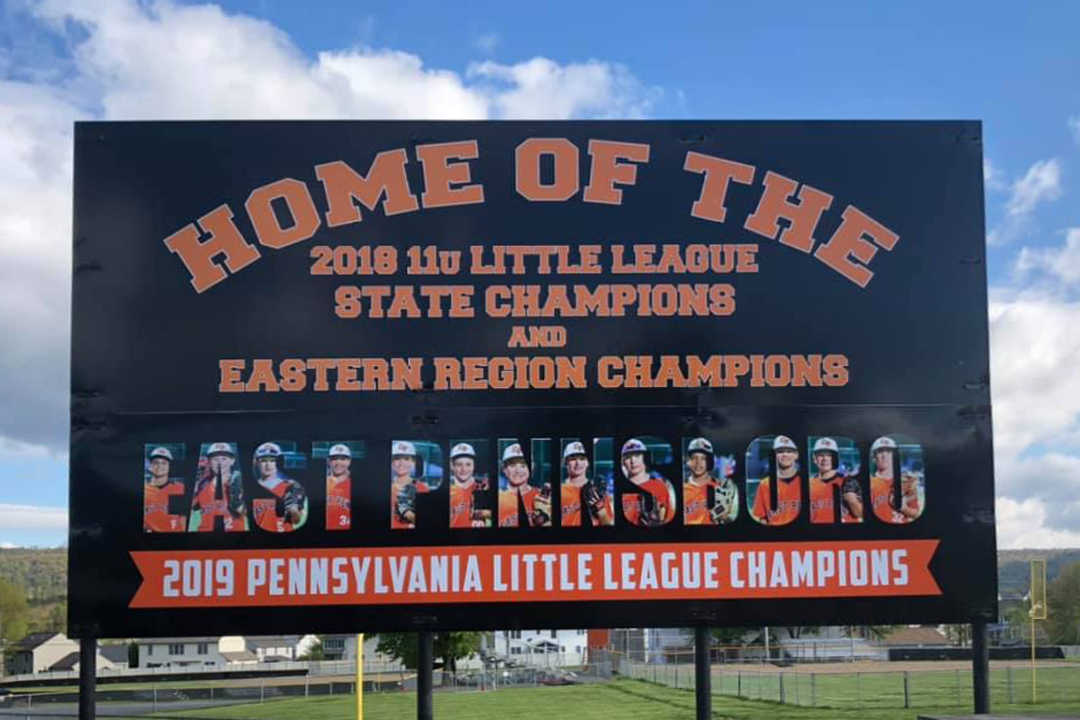The billboard stands prominently on four round black poles and features multiple lines of celebratory text. At the top, large black text on an orange banner proudly announces "Home of the 2018 11U Little League State Champions and Eastern Region Champions." The name "East Pennsboro" is creatively displayed in large block letters, each filled with photographs of the triumphant baseball team members, who are shown wearing their orange uniforms. Beneath, a contrasting red banner with white text declares them the "2019 Pennsylvania Little League Champions." Beyond the billboard, a row of lush, green baseball fields—neatly trimmed and enclosed by chain-link fences—extends into the background. The scene is set under a bright blue sky dotted with white clouds, adding to the vibrant and celebratory atmosphere.